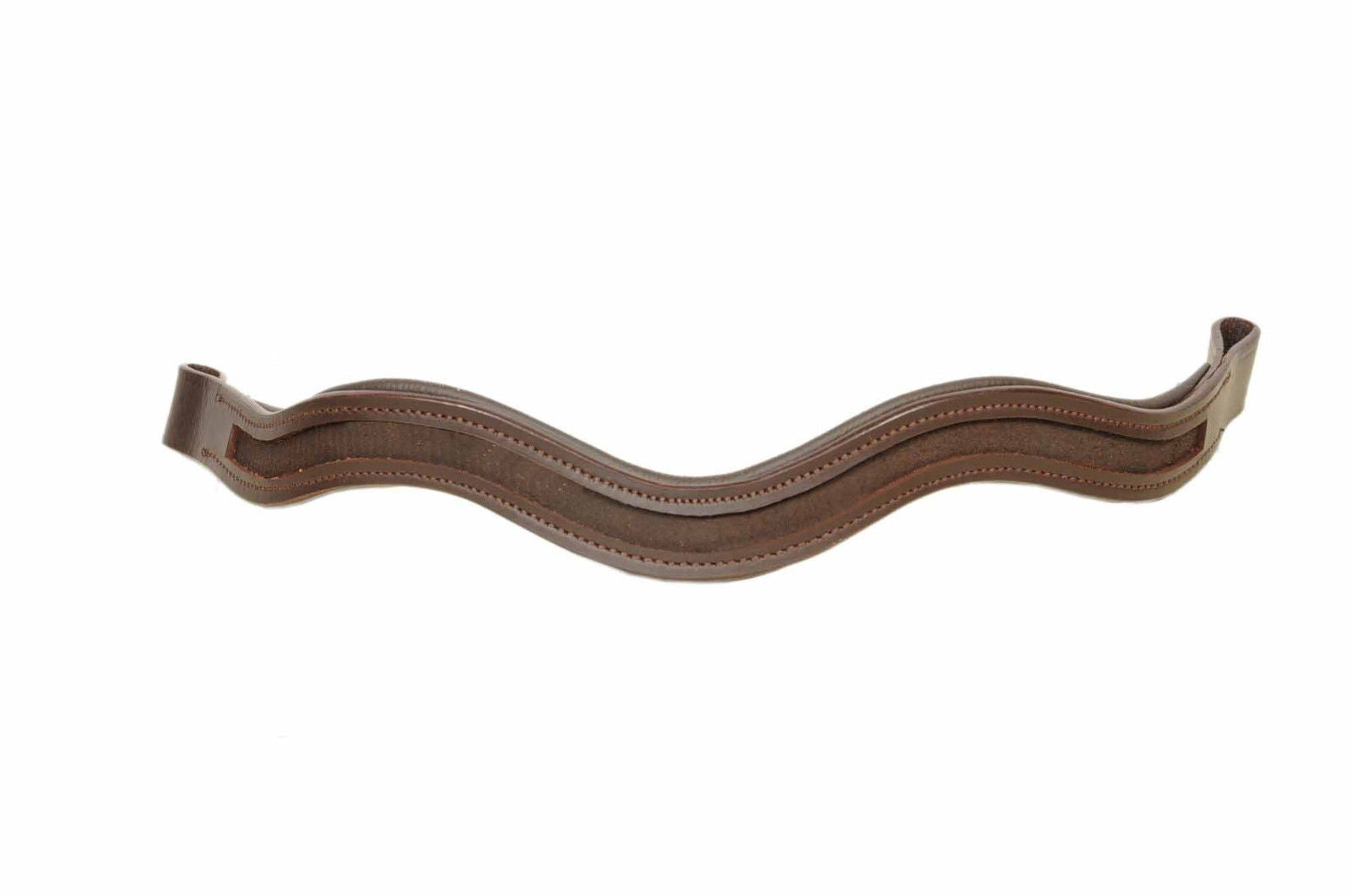The image depicts a brown leather strap, possibly used as a shoulder strap or for carrying purposes. The strap lies horizontally against a fully white background, creating a perception that it is floating in midair. The strap features two loops at either end where the leather is sewn behind itself to form attachment points. These loops contain circular holes through which an item can be threaded for attachment. Running down the center of the strap is an indented groove that extends from one end to the other, flanked by meticulously small stitches. The stitching, which matches the leather in color—perhaps slightly lighter—highlights the craftsmanship involved. The strap has several curves, accentuating its natural bends and adding to the intricacy of its design.